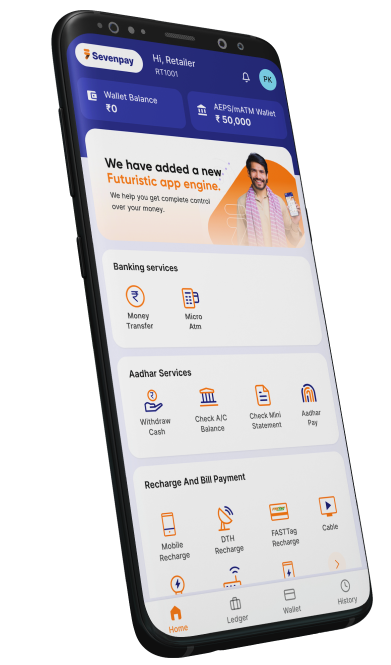The image displays a smartphone screen showcasing a financial application interface named "7Pay." At the top of the screen, a greeting reads, "Hi Retailer," followed by an ID labeled "RT-1001." A white bell icon indicates notifications, and a circular icon with the initials "PK" is also visible.

The wallet is bifurcated into two segments: a main wallet balance of 0 and an AEPS/MATM wallet balance of 50,000. Below these details, there is an image of a man smiling while holding a phone. Beneath the image, text announces the addition of a new futuristic app engine and promises users complete control over their money.

The interface offers various banking services, including money transfers, microATM, and Aadhaar-based services such as cash withdrawals and balance checks. Options for viewing mini-statements are also available. Additional sections cover recharge and bill payment options, including mobile and DTH recharges, as well as cable services. These features are represented by a variety of orange icons, each typically depicting a small screen relevant to the action they represent.

At the very bottom of the screen, there are four navigational sections: Home, Ledger, Wallet, and History.